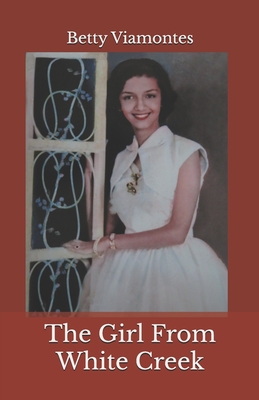This image appears to be a color photograph of a book cover. The background of the cover is a maroon or dark red color, with the title "Betty Villamontes" written in white text at the top and "The Girl from White Creek" in white text at the bottom. In the center of the cover is a photograph of a smiling woman, who seems to be in her mid to late 20s. She is facing the camera, wearing a sleeveless white dress with a poofy skirt and a small bolero jacket-like cape. The woman has short, dark hair and is adorned with bright red lipstick and a necklace with bead-like ornaments. Her left hand is resting on a small, wooden decorative shelf or trellis, while her right hand is positioned behind it. The overall style suggests a mid-1950s era aesthetic. There are no other people in the photograph.